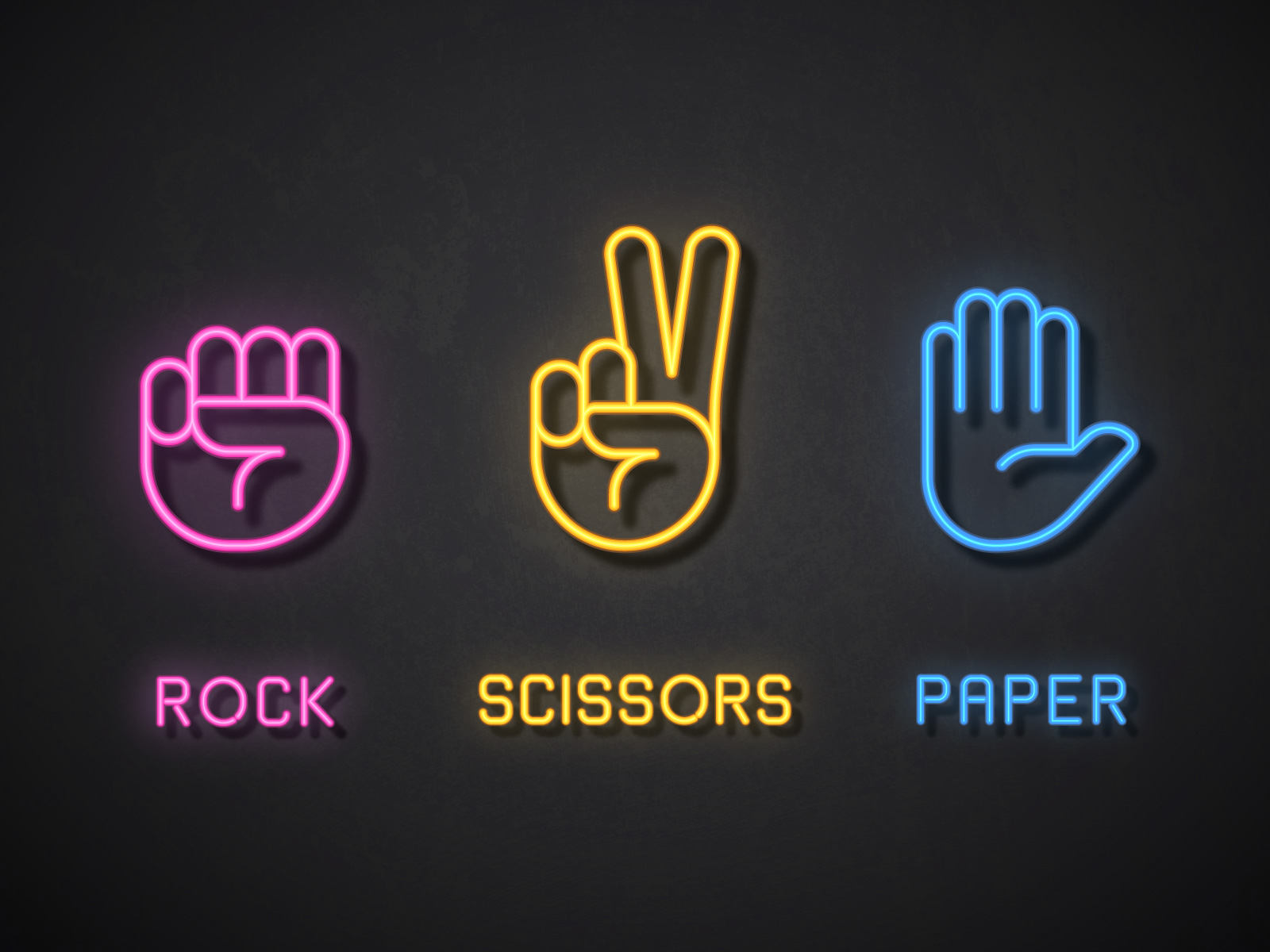The illustration features three vibrant neon signs set against a dark gray to black background. Each sign displays a different hand gesture associated with the game "Rock, Paper, Scissors," along with corresponding text that matches the color of the neon light. From left to right, the first sign is a bright pink fist representing "Rock," with the word "Rock" written underneath in matching neon pink. The middle sign, in vivid yellow, shows a hand making the peace sign for "Scissors," with "Scissors" written below. The third sign on the right is a luminescent blue, depicting an outstretched hand symbolizing "Paper," with "Paper" written beneath it in the same shade of blue. The neon signs are all positioned side by side, contributing to a dynamic and eye-catching composition.